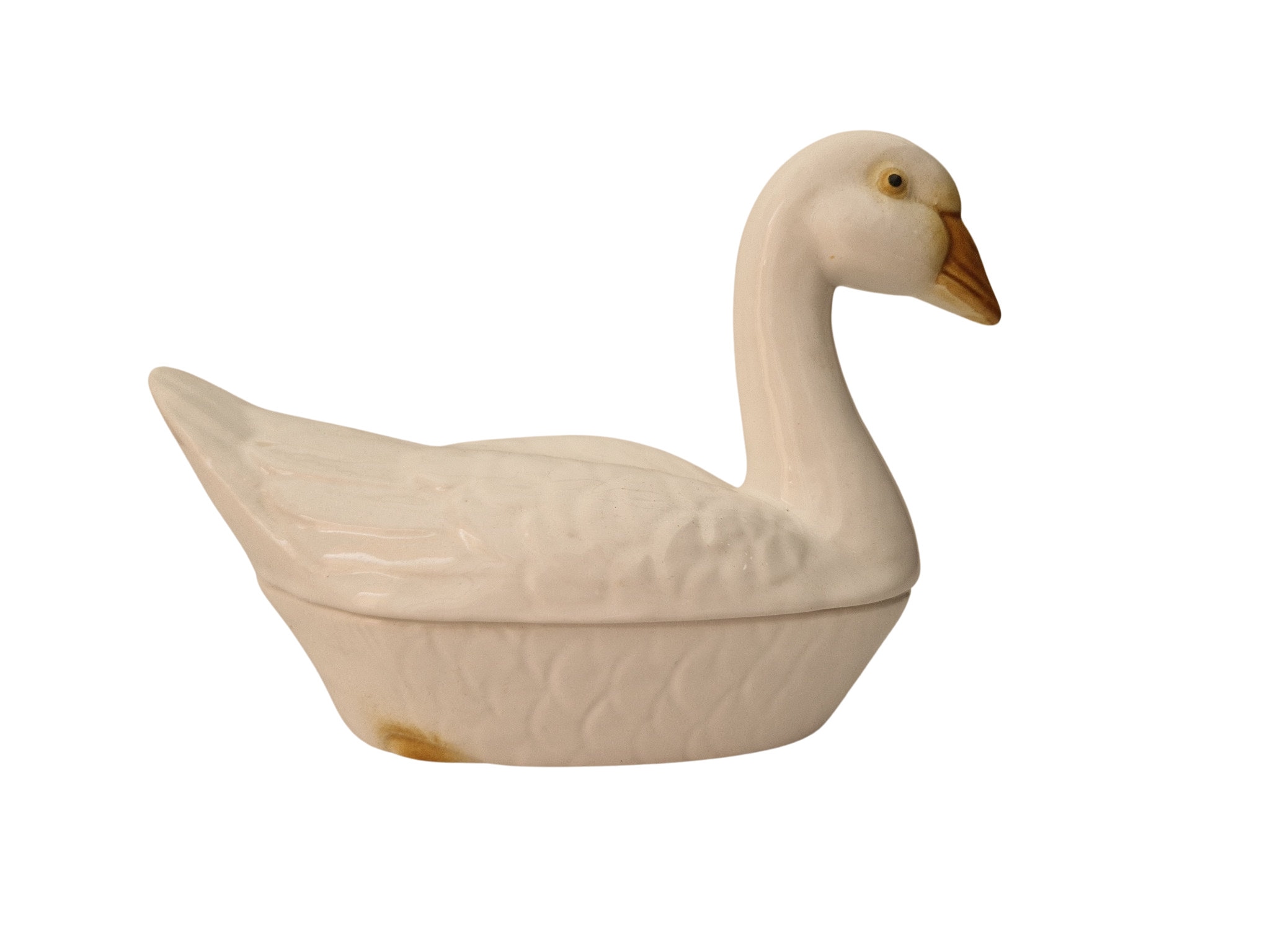A detailed color photograph showcases an intricately designed ceramic or porcelain baking dish, artistically crafted in the shape of a swan. The swan, potentially also interpreted as a duck, is oriented to face the right. Notably, it features a distinctive yellow eye and a yellow beak. The swan's back is gracefully arched, while its tail feathers elegantly curve upwards. At the bottom left corner of this sculpture, a yellow section probably represents a foot, adding to the lifelike detail. The surface is meticulously etched to replicate feathers, imparting a textured appearance. The glossy finish, particularly evident on the neck and back, highlights its reflective quality. A subtle seam suggests that the top section of this sculptural piece can be lifted off, possibly transforming it into a functional item for serving or baking.